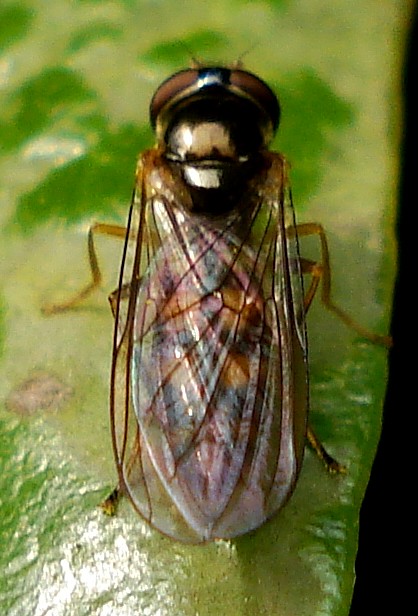This extremely close-up photograph showcases a predominantly brownish insect, likely a bee or beetle, resting on a shiny green object, which appears to be a leaf. The insect's body features a mix of brown, orangey tones and possibly yellow and black stripes, consistent with the description of a bee. Its head and bulging eyes are visible from the back, accompanied by small antennae and extended legs on both sides. The insect's translucent, folded wings glisten, subtly revealing the intricate structure beneath. The green surface it rests on contrasts with the solid black background framing the image.